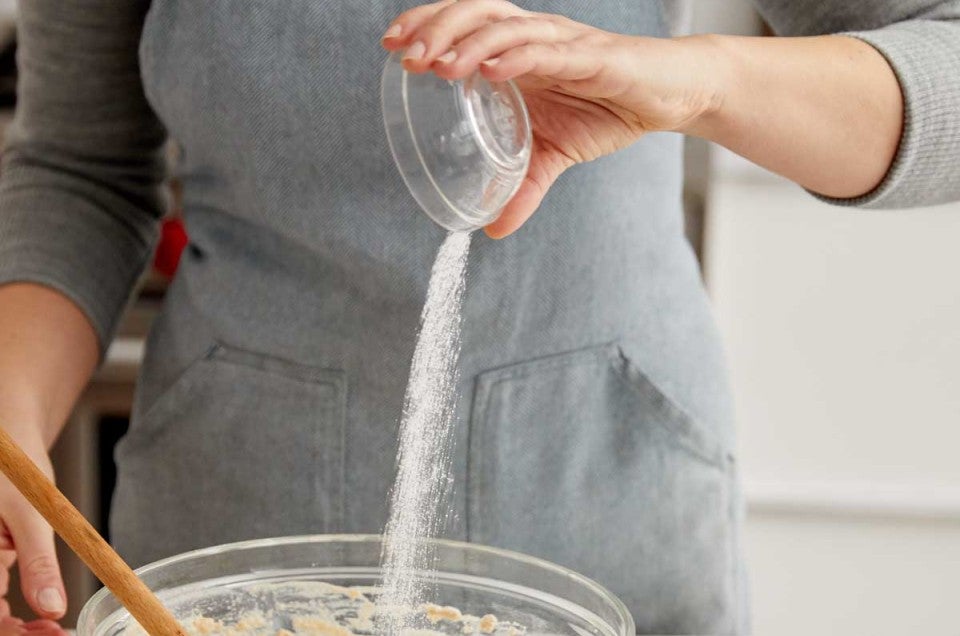In this indoor kitchen scene, a woman, whose identity is obscured from the chest down, is captured in the act of cooking. She appears to be Caucasian and is dressed in a gray sweater with long sleeves, which are rolled up, and is accessorized with an apron featuring two pockets. A small red ribbon is tied around her waist. She is pouring sugar, or possibly salt, from a small, clear plastic bowl into a larger mixing bowl below, which contains some orange-colored dough or mixing material and a wooden spoon. The background is a blurred kitchen setting with a white wall or refrigerator in the far right corner of the image. The focus of the photograph is on the woman's precise actions and the ingredients she is using.